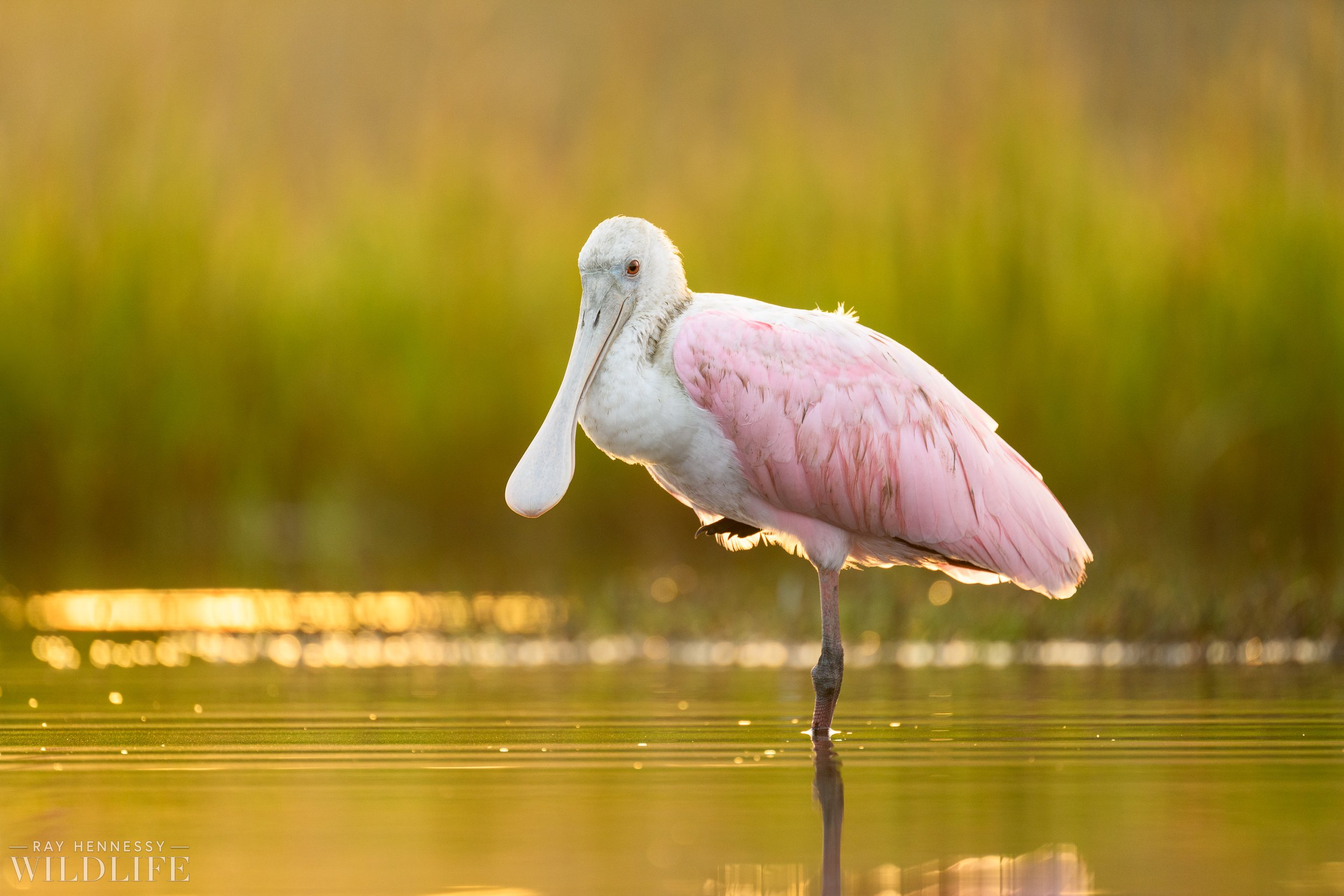A horizontal, close-up photograph captures a bird standing in shallow, yellowish-green water. The bird, which appears to be a flamingo or a crane, has a slender, oblong beak that rounds at the end and is a whitish-pink color. The bird's head is small with a notable red dot in its eye. Its body is primarily white with strikingly vibrant pink feathers on its back and wings. One of its long legs is submerged, with the water reaching just below the knee joint, while the other leg is tucked underneath its body, with just a hint of the foot visible. The neck is retracted, making its length indiscernible. In the blurred background, a shoreline is faintly visible, possibly with a sidewalk, trees, and weedy undergrowth, creating an environment that accentuates the bird's elegant form as it stands serenely, seemingly alert and looking towards the viewer.